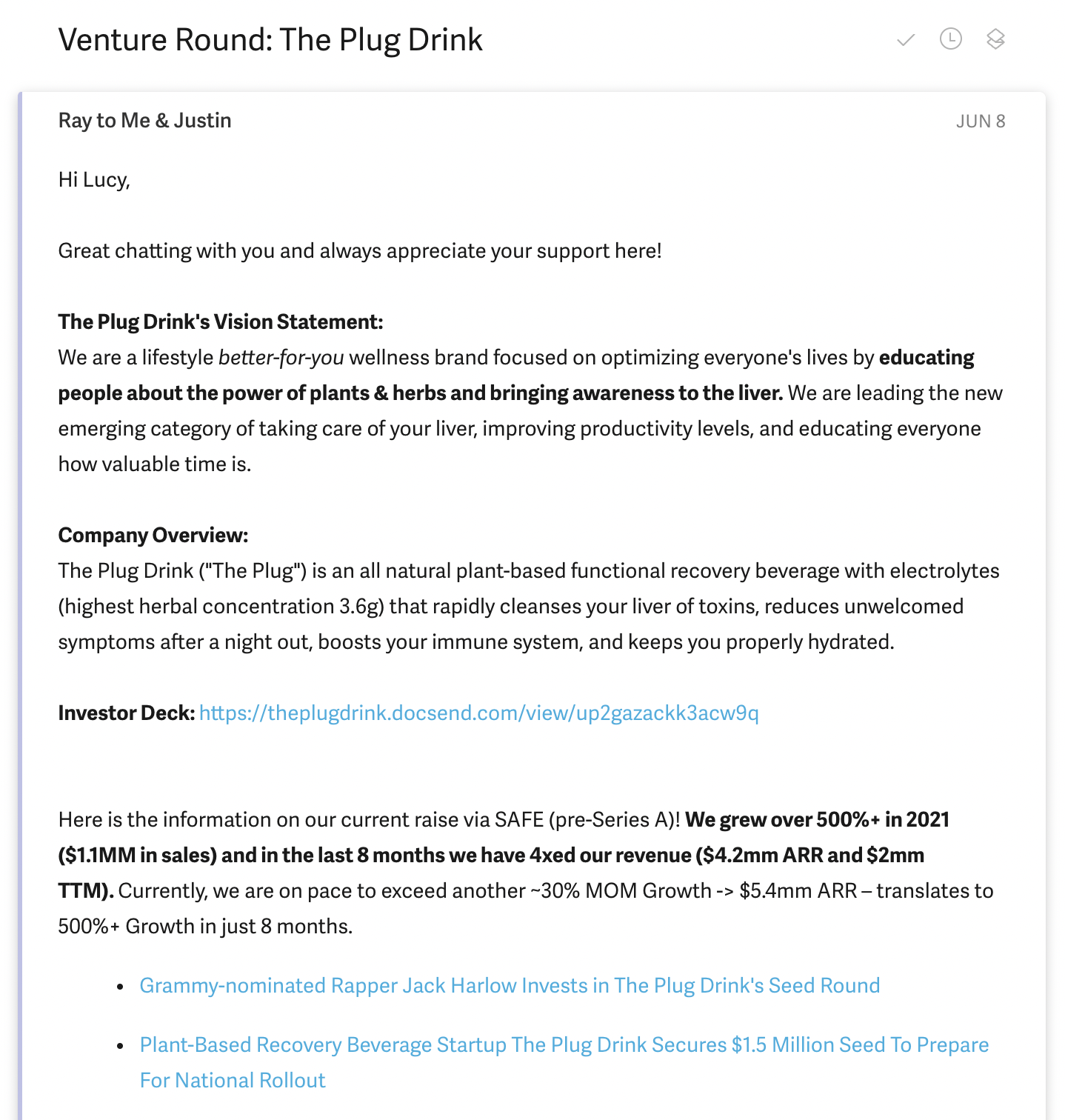Caption: 

The image features an email from The Plug Drink, a wellness brand dedicated to optimizing lives through the use of plant-based and herbal remedies. In the email, founders Ray and Justin greet Lucy and express their appreciation for her support. The letter highlights The Plug Drink's mission to educate people about the benefits of herbs and plants, particularly their importance for liver health. 

As a company overview, The Plug Drink is introduced as a plant-based functional recovery beverage enriched with electrolytes and a high herbal concentration (3.6 grams), designed to rapidly cleanse the liver, alleviate symptoms after a night out, boost the immune system, and improve hydration. An impressive company performance is presented, including a 500% growth in 2021, sales of $1.1 million, and a recent fourfold increase in revenue, reaching 4.2 million in Annual Recurring Revenue (ARR) with a 30% month-on-month growth. The company aims to continue its impressive trajectory with a projected 5% growth over the next 8 months.